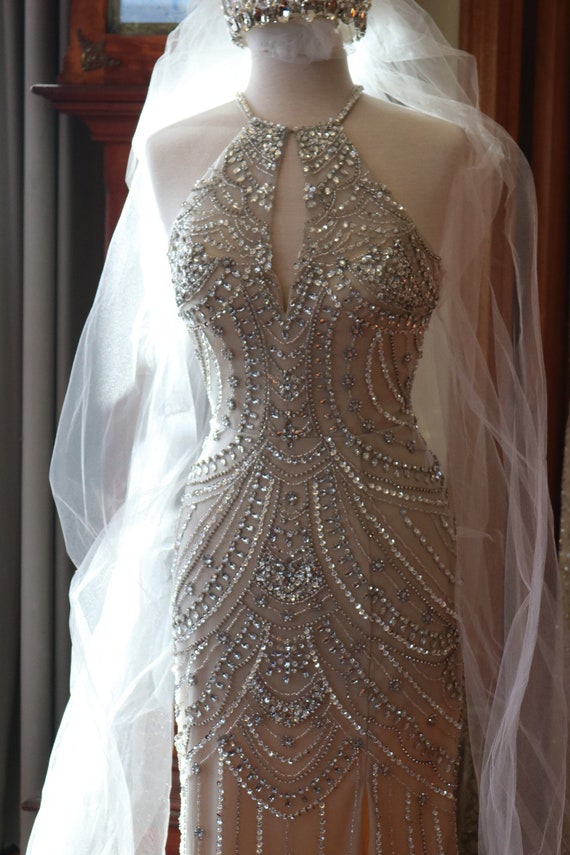This vertically oriented photograph showcases a stunning, sleeveless wedding gown displayed on a mannequin. The gown appears to be a light, possibly cream or champagne color, adorned with intricate, curved patterns of sequins and rhinestones that create a shimmering, ornate effect, indicative of its high-end nature. The dress features a scoop neck design and is complemented by a luxurious, floor-length, white silk veil. The veil is elegant and sheer, adorned with a band of stones, crystals, and beads, possibly forming a tiara or crown-like headpiece on the mannequin. The scene includes some wooden furniture in the background, indicating that the display is set inside a room, with the view captured from about the knees up to eye level.